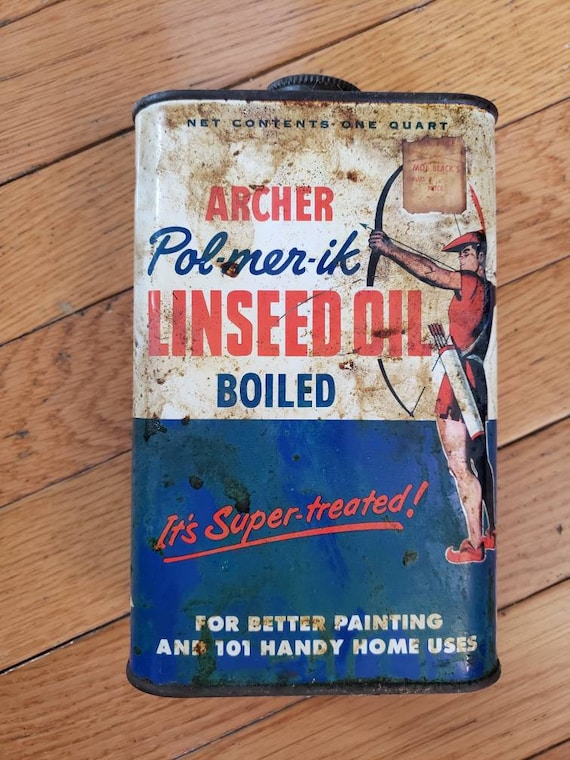This photograph features an old, rusted metal container of linseed oil, prominently labeled "Archer Polymer Linseed Oil, Boiled." The can has a screw cap on top and is divided into two colored sections: the top half is white, and the bottom half is medium blue. The text on the can is in red and blue. At the very top, in blue text, it reads "Net Contents 1 Quart," with a faded sticker below it that says "Mod Black." Beneath that, "Archer" is written in bold red letters, followed by "POL-MER-IK" in blue script, "Linseed Oil" in bold red letters, and "Boiled" in blue. The bottom blue section reads "It's Super Treated" in red script, underlined, and "For Better Painting and 101 Handy Home Uses" in bold white letters. 

On the right-hand side, there is an image of an archer dressed in a Robin Hood-like outfit with a red top, short skirts, a red cap with a feather, and red shoes but no leggings. A strap around the archer’s waist holds a quiver filled with arrows, one of which is drawn in a black bow aimed at the word "Archer." The can is old and stained, and it rests on a wooden plank floor.